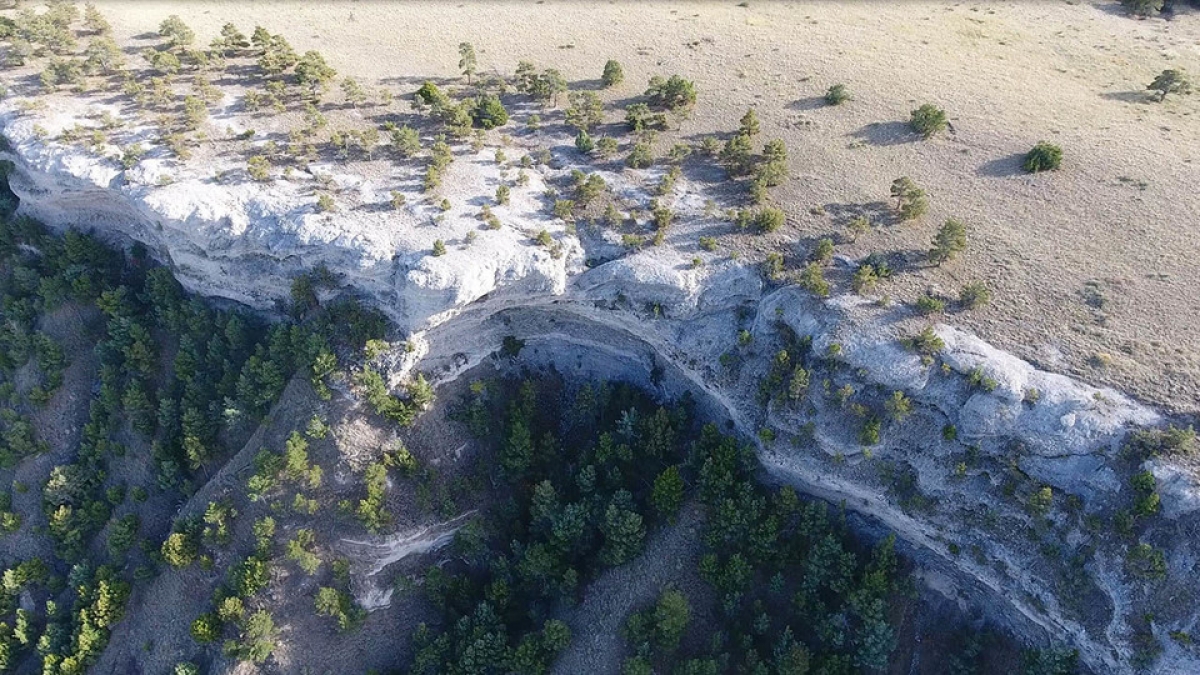The image features an aerial view of a remote, arid landscape dominated by a striking geologic formation. At the center, a flat-topped mesa or plateau rises above the surrounding terrain, its white-cliffed edges—possibly chalk or limestone—creating a sharp, contrasting boundary. Sparse shrubbery and scattered evergreen trees adorn the top of the plateau, while more densely packed coniferous trees extend down the rocky, brown slopes. The play of sunlight casts stark shadows, highlighting the jagged edges of the cliffs and the uneven terrain below. The entire scene is devoid of any signs of human civilization, emphasizing the untouched, wilderness nature of the area, with large swathes of barren soil and patches of white dirt accentuating the rugged beauty of the landscape.